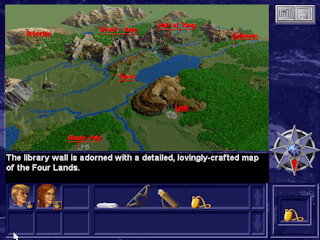This image is a detailed screenshot from a computer game. The main feature of the top half of the screen is an overhead, topographical map that displays a diverse outdoor area, including mountains, wooded forests, streams, lakes, and possibly caves or towns, highlighted with red labels for identification. The map also features some character names, including "Leah." Underneath this map, a black panel with white text reads, "The library wall is adorned with a detailed, lovingly crafted map of the four lands," suggesting it could be a clue for solving puzzles or advancing in the game.

The lower half of the screen includes artistic illustrations of two characters: a blond male and a red-headed female, both facing right. Next to these figures is a rectangular area displaying objects obtained during gameplay, such as eyeglasses and a pocket watch. To the right side of the map, a starlight compass with a prominent red star point at 6 o'clock is visible, likely serving as a navigation tool. The lower rectangular area and the vertical panel beside the map are navy blue or black, framing the intricate details and elements of the game interface.